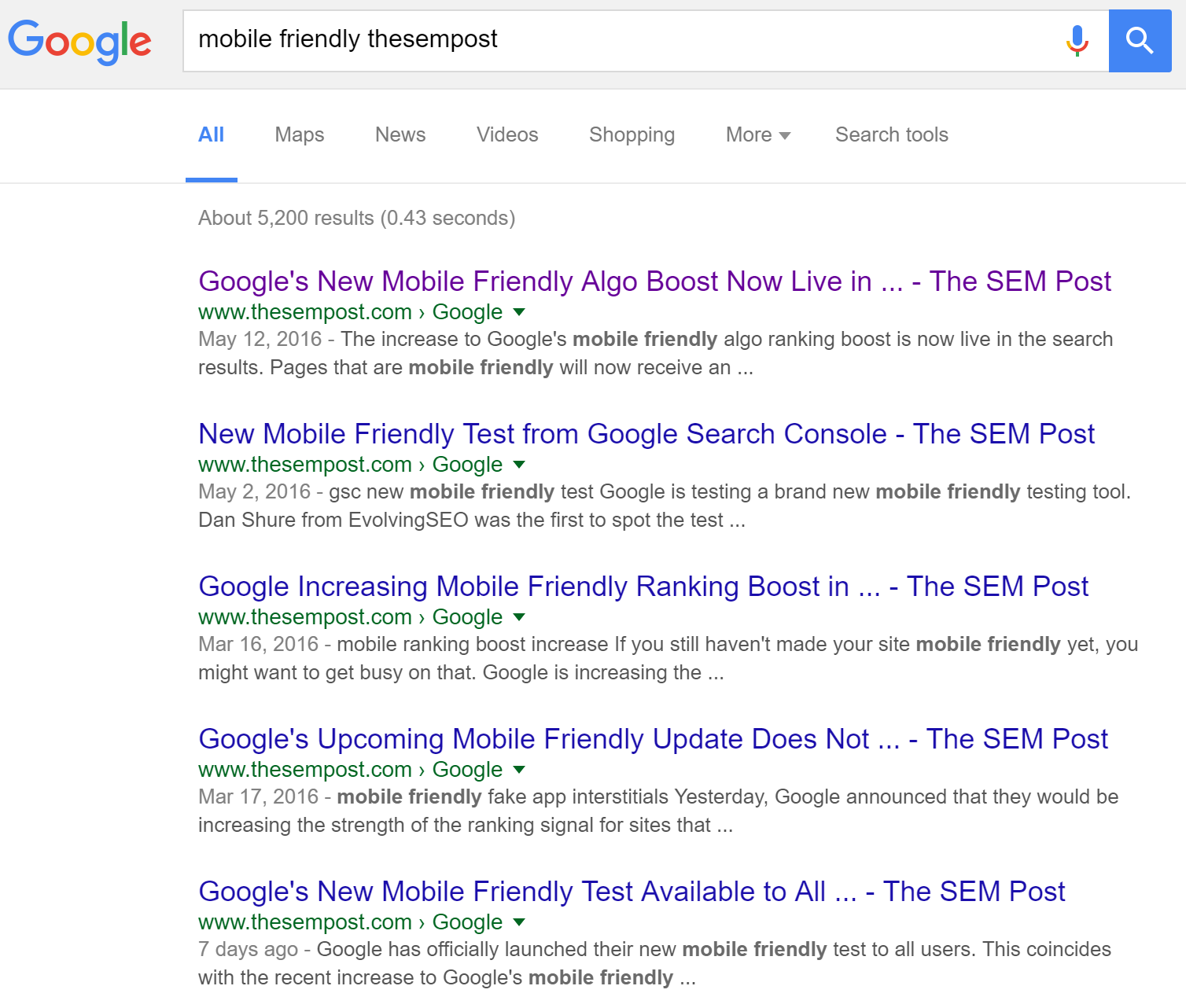This is a screenshot of a Google web search. At the top, there is a gray banner with "Google" displayed on the top left. Next to it, there is a search bar with a microphone icon and a search icon to the right. Below this banner, the web page has a white background and features a row of horizontal categories labeled All, Maps, News, Video, Shopping, More, and Search Tools, with "All" highlighted.

The search term "mobile-friendly" is entered in the search bar. The search results page displays a list of links with the top result showing "Google's new mobile-friendly algo boost now live" from "The SEM Post,” although it appears as a single word due to a typing error. This particular top result is colored purple, indicating it has been clicked on before, while the remaining search results are in blue. There is a full page of search results presented below the initial top result.